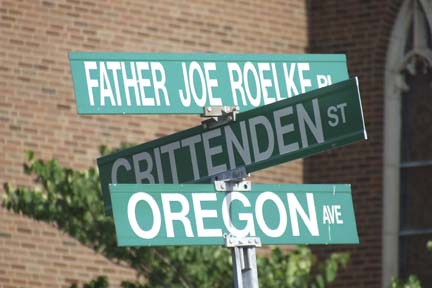The image depicts a multi-street corner with a post that supports three green street signs with white lettering. The top sign reads "Father Joe Roelke Place," parallel to the bottom sign, which reads "Oregon Avenue." The middle sign, positioned perpendicular to the bottom sign, reads "Crittenden Street." The post is steel with a riveted bracket at the top. In the background, there is a tree and a large, multicolored brick building, possibly a church, illuminated by sunlight. On the right side, barely visible, is the edge of a white window or structure casting a shadow, creating a contrast between the brightly lit left side and the darker right side of the image.